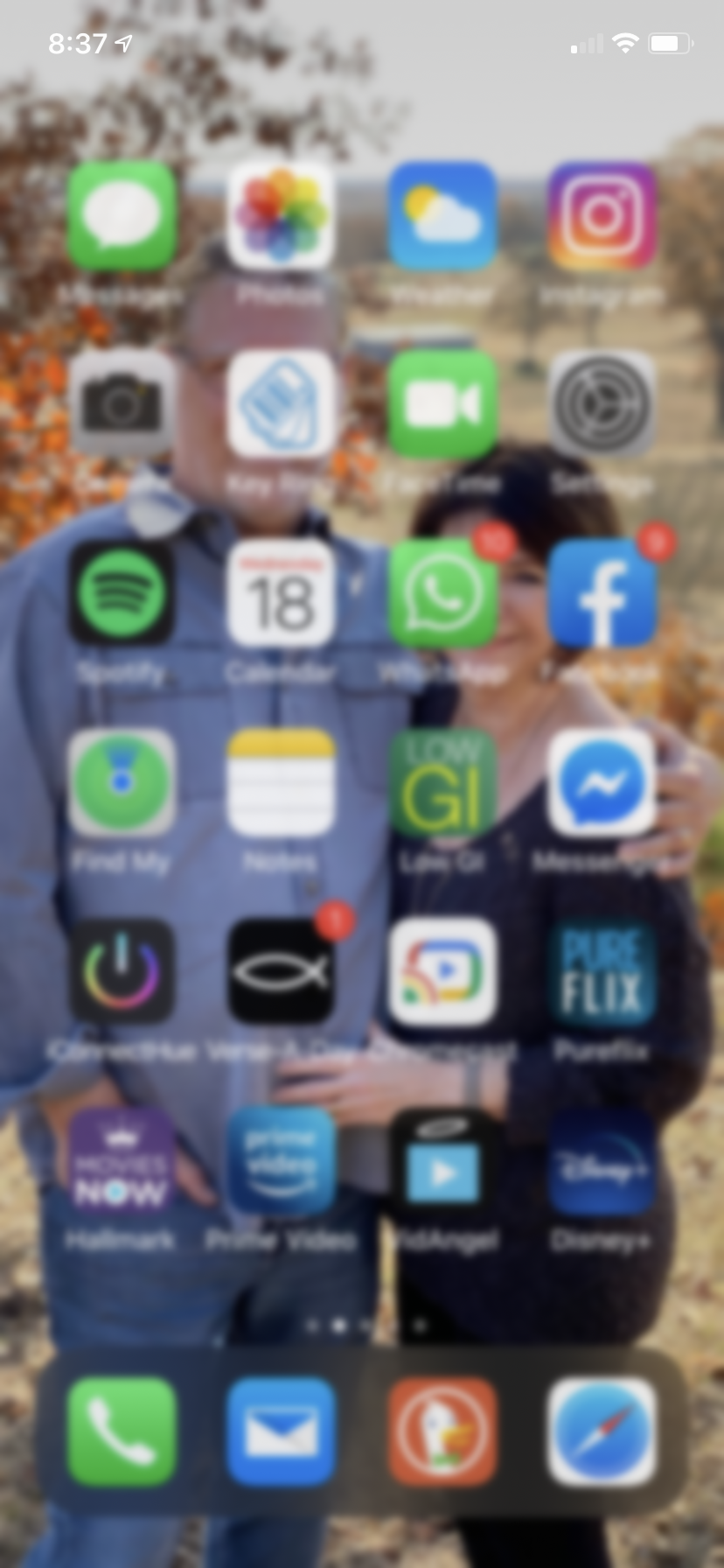A blurry image of what appears to be an iPhone screen is depicted. In the top left corner, a white font displays "8:37" with a small arrow pointing to the upper right. The upper right of the screen shows one bar of cell service, full Wi-Fi bars, and approximately 80% battery life, all indicated in white.

The background image features a slightly discernible scene of a man and woman holding each other. The man is dressed in a blue button-up shirt and blue pants, with one hand in his pocket and the other wrapped around the woman. The woman, sporting brown hair, is clad in a blue shirt and black pants. The backdrop of the image suggests an autumnal forest setting, though details are unclear due to the blurriness.

Despite the overall blur, the phone's apps and icons are somewhat recognizable. The apps at the bottom of the screen include a green phone icon, a blue mail icon, the DuckDuckGo logo, and the Safari logo.

Arranged from top left to bottom right, the apps include:
1. Messenger
2. Photos
3. Weather
4. Instagram
5. Camera
6. An unidentified blue glove icon
7. A green camera icon
8. Settings wheel
9. Spotify
10. Calendar
11. An icon with a text bubble and a phone
12. Facebook
13. Find My
14. Notepad
15. An icon with "low GI"
16. Messenger
17. A power button in rainbow colors
18. An icon with a fish on a black background
19. Google Play
20. PureFlix
21. Movies Now
22. Amazon Prime
23. A blue play button with a halo above it
24. Disney Plus